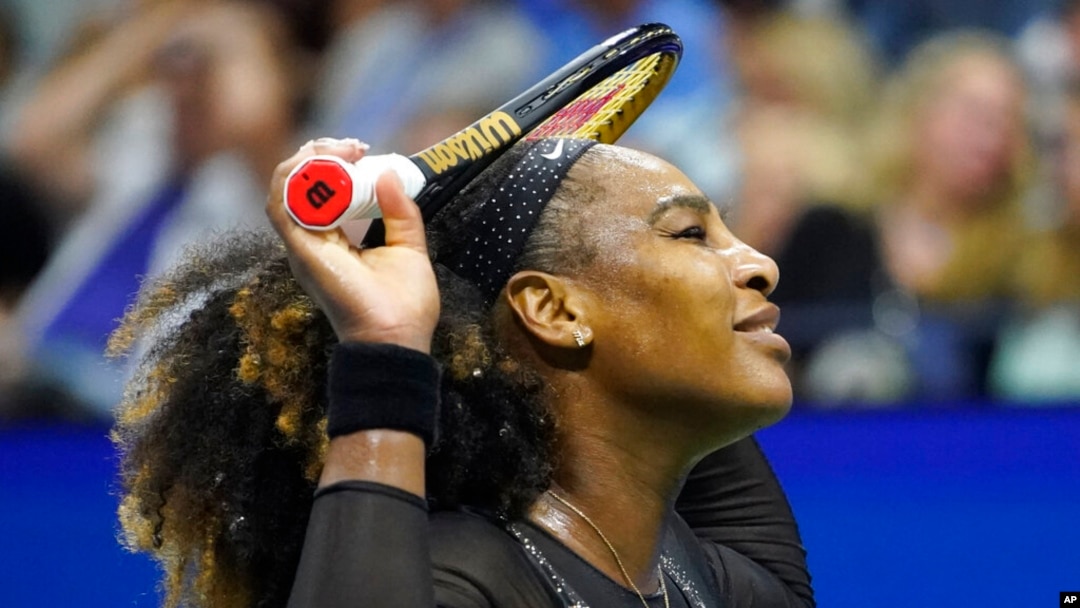This detailed image captures a close-up of Serena Williams, the iconic tennis player, during a strenuous moment at a tennis tournament. The photograph focuses on Serena from the shoulders up, highlighting her side profile as she faces right with her eyes closed and mouth partially open, revealing her teeth—a look that suggests extreme fatigue or pain. Her hands are raised above her head, holding a black Wilson racket with yellow webbing and a white and red handle, which rests atop her head. She is adorned in a skin-tight black long-sleeved shirt, a black and white spotted Nike headband, a black wristband, a small earring in her right ear, and her long black hair flows out to the left behind her. The backdrop features a blurry blue wall at the bottom and indistinct spectators filling the stands. The scene is subtly stamped with "AP" in the bottom right corner.